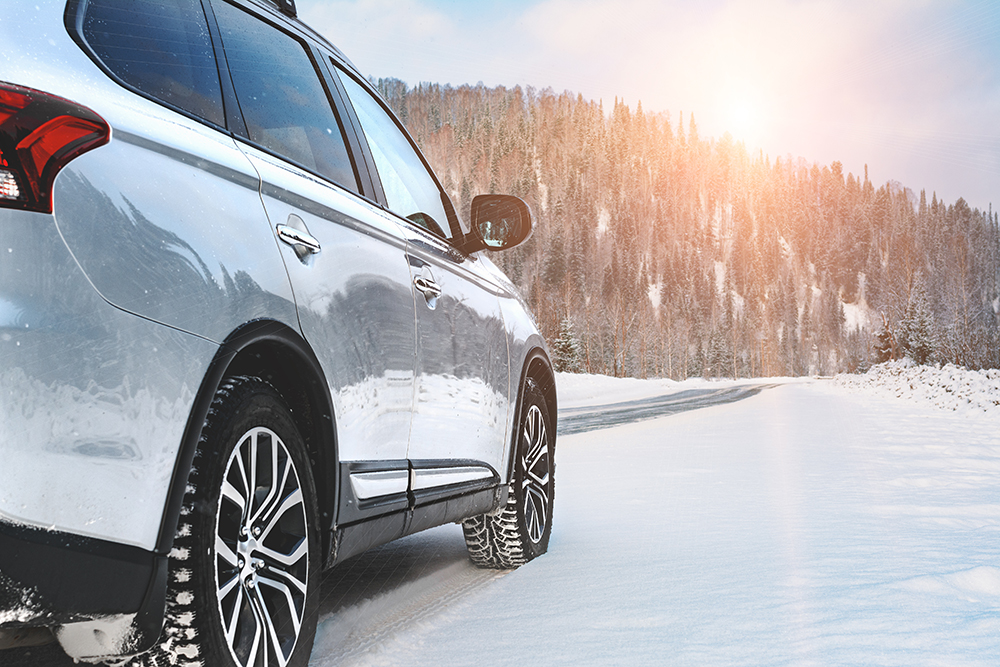In this detailed photograph, a silver or light blue four-door car with black snow tires is parked on the snowy shoulder of an asphalt roadway. The car is positioned centrally, angled from the back-left side, making part of its rear and side visible. The serene winter scene is dominated by a snow-clad mountain in the background, which is densely forested with green pine trees. The mountain rises up, creating a natural barrier. Above, the sky is dreary yet vibrant where the sun, yellow in its hue, peeks through a veil of clouds, casting a soft light over the landscape. The roadway beside the parked car is mostly clear of snow, suggesting recent plowing or traffic, though the surrounding snow appears to be an inch deep. The whole scene evokes a picturesque, peaceful alpine setting, possibly hinting at a ski destination nearby.